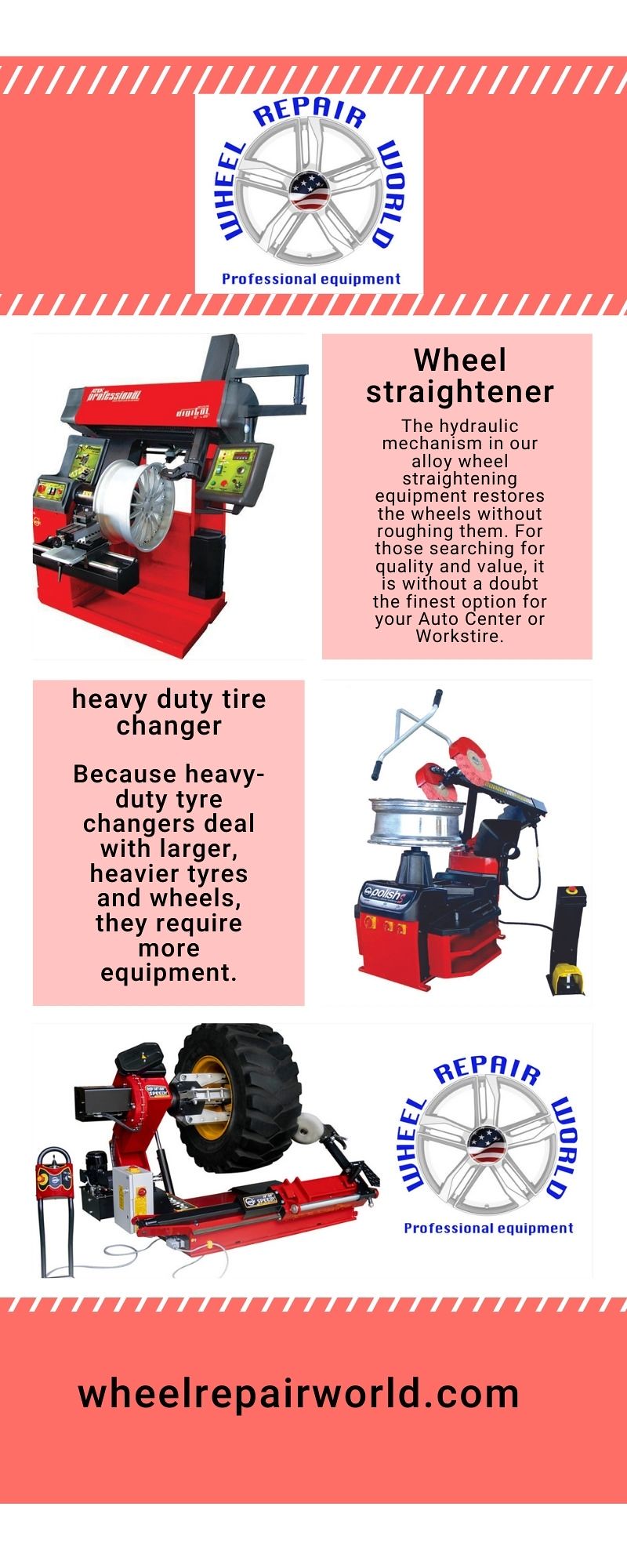This advertisement for Wheel Repair World features a meticulously designed promotional piece, combining photographs, illustrations, graphic design, and typography. The image is in portrait orientation with a narrow format, framed at the top and bottom by horizontal bands of dark peach color with white hand stitching.

At the top center, within a white square, is the Wheel Repair World logo, showcasing a car wheel in gray line art with a red, white, and blue hubcap, and surrounded by the name "Wheel Repair World" in blue writing. Below the logo is a series of professional wheel repair equipment.

To the left, beneath the main logo, is a red and black machine working on a silver car wheel. To its right is a salmon-colored box with black text that reads "Wheel Straightener." This description highlights the hydraulic mechanism of the alloy wheel straightener, emphasizing its ability to restore wheels without causing damage and touting it as the finest option for quality and value at an auto center workplace.

Further down, on the left, there is another box with the title "Heavy Duty Tire Changer" in black font on a pink background, accompanied by an image of the tire changer machine in red and black, holding a silver wheel.

To the right of these machines and texts, there is another piece of equipment depicted — a tire balancer — aligned with the branding aesthetics.

At the very bottom of the advertisement, the Wheel Repair World logo reappears on the right, mirroring the top logo, and to the far right is the website URL "wheelrepairworld.com" in dark lettering. This cohesive visual presentation showcases the high-quality wheel repair equipment available from Wheel Repair World, blending photographic representationalism with illustration and compelling graphic design.